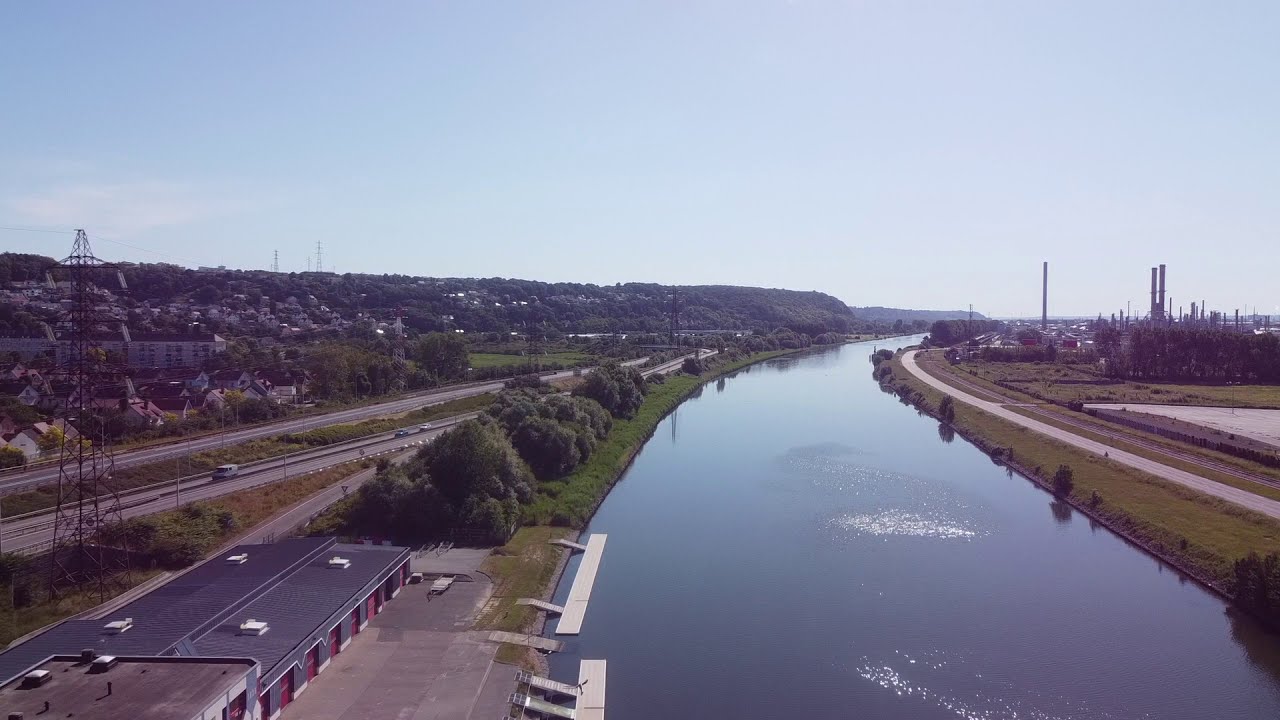In this detailed aerial image, we see a large and clear river or canal flowing from the bottom right towards the center of the image. The water is relatively calm and may have some white waves or disturbances in the middle. On the right side of the river, there is a grassy area with a cement walkway or pathway adjacent to a field. Near the bottom right corner, there's a building resembling a storage unit with red or orange doors and a black roof topped with white fixtures. Nearby, power poles and lines are visible. 

To the left of the river, in the lower left corner, there is a robust cluster of trees and grass, accompanied by a building that appears to be an industrial processing plant or another storage facility. This structure is positioned near what looks like a boat ramp. Further upward, we see a four-lane highway with a few cars on it, running parallel to the river. 

In the background, there are several buildings and possibly a residential area. Prominently, there is one tall skyscraper and two smaller buildings clustered together to the right. There are also smokestacks or chimneys visible near these buildings. The sky above is mainly clear with a few clouds on the back left side, suggesting a bright, sunny day. The image captures various colors including brown, black, red, green, tan, gray, and blue, painting a vibrant and detailed scene.